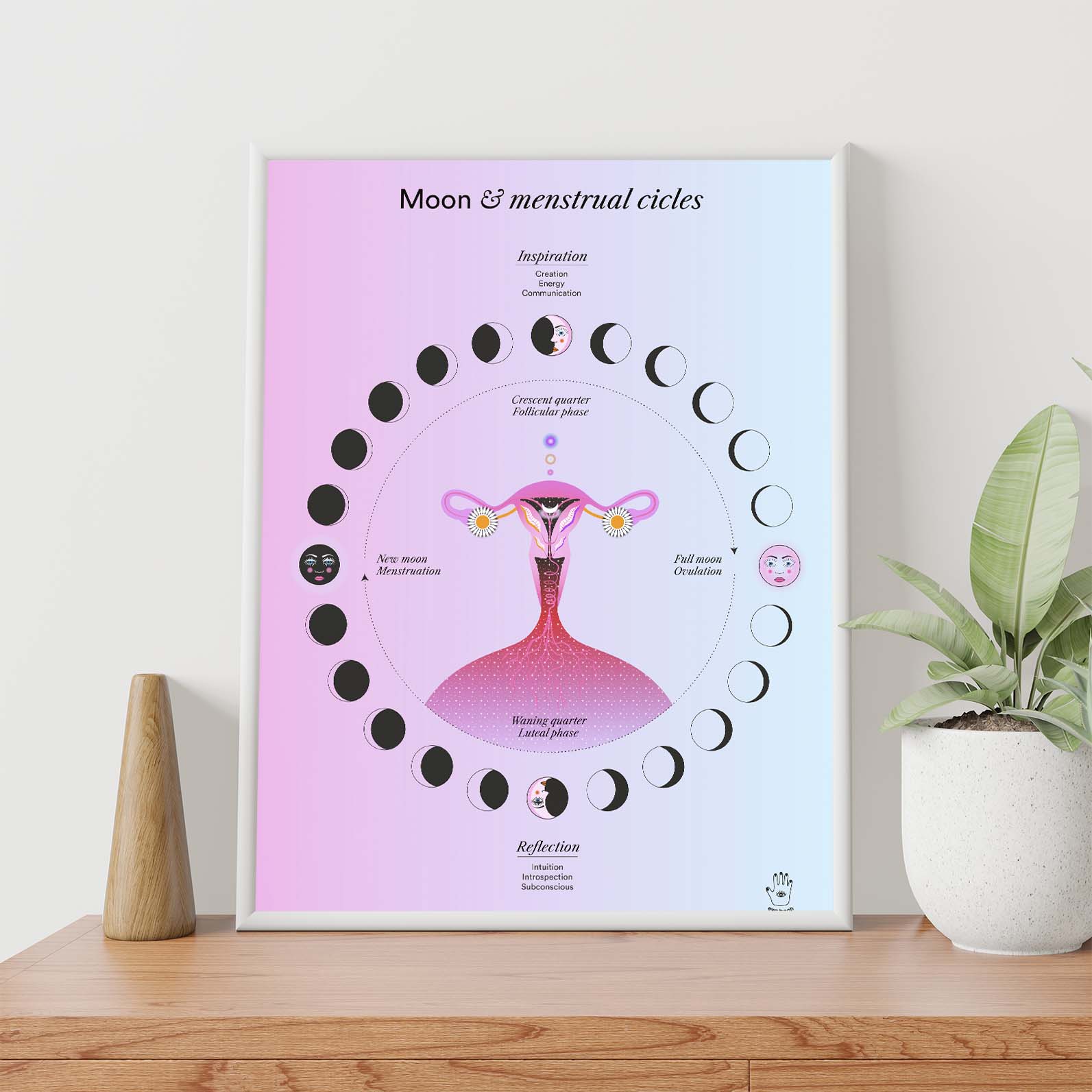The photograph is a professionally taken color image, seemingly crafted for an advertisement or informative poster. Central to the composition is a white-framed print with a gradient background transitioning from pink on the left to blue on the right. The top of the poster prominently features the title "Moon and Menstrual Cycles," although "cycles" is misspelled as "cicles." The focal point of the poster includes a detailed diagram of a woman’s reproductive organs encircled by the various phases of the moon. Key words such as "inspiration," found at the top, and "reflection," at the bottom, are textually highlighted within the design.

The soft lighting and professional setup draw attention to the framed print, which is placed on a long wooden table. The table extends from the bottom left to the bottom right of the image, beneath a backdrop of a large white wall. Positioned to the left of the framed print is a pyramid-shaped wooden sculpture, and to its right, a white clay pot houses a plant with lush green leaves and visible soil. The overall setting is clean and serene, showcasing the poster in a well-balanced and contextualized environment.